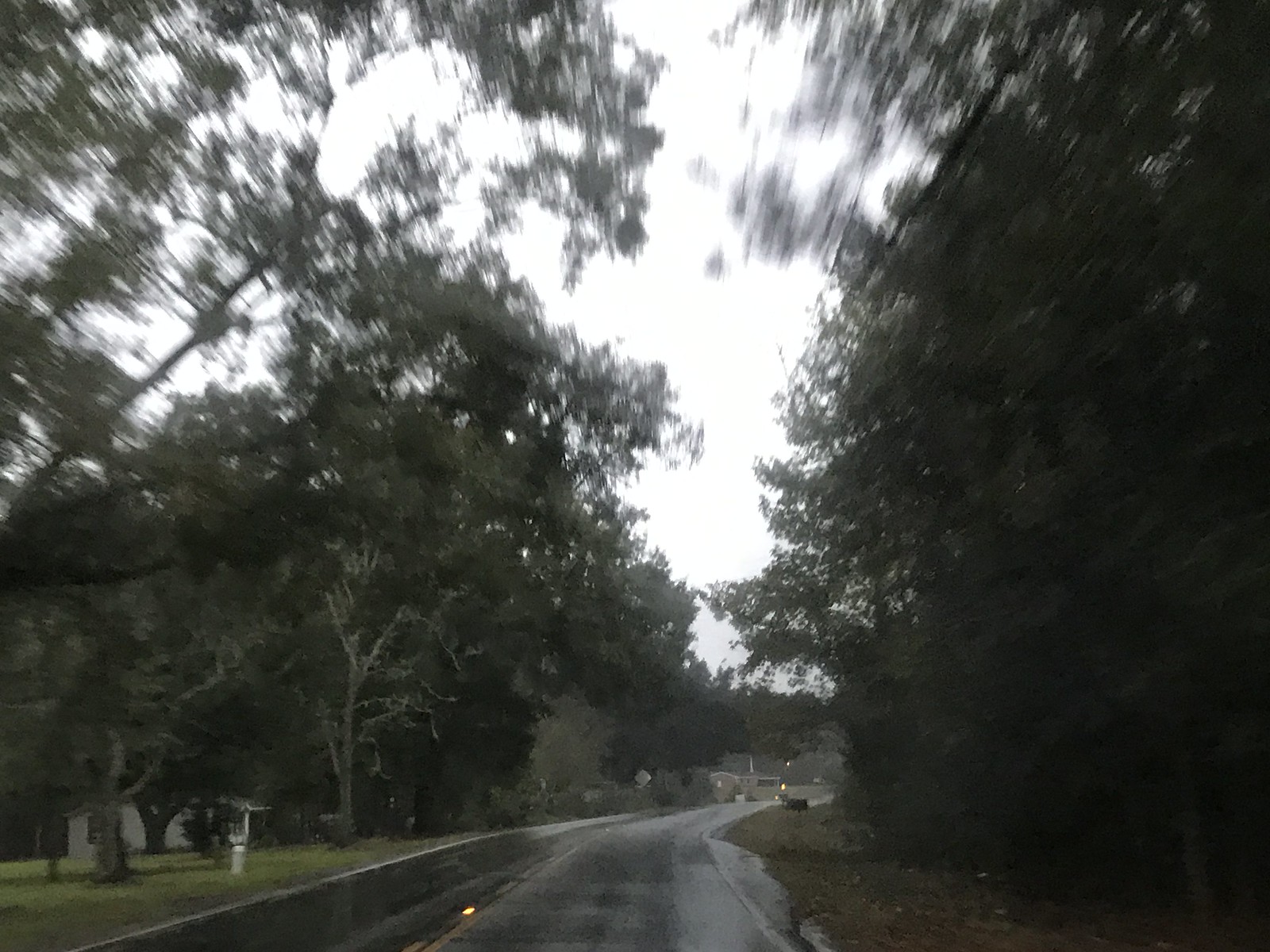A serene, dimly-lit street stretches ahead with two lanes vanishing into the distance. On the left side in the background, a quaint house peeks through the shadowy edges, partially obscured by a dense canopy of trees. The right side of the street is enveloped by tall trees with lush, green foliage, allowing only faint beams of light to seep through at the fringes. More trees line the opposite side, contributing to the overall darkness of the scene. In the top left corner of the image, some leaves appear blurred, adding to the mysterious ambiance. Towards the bottom left, more details emerge: a mailbox stands sentinel amid the greenery, and the house reappears, framed by the shadows of the towering trees. The photograph exudes a moody, subdued palette dominated by shades of gray, green, and black, enhancing its tranquil and introspective atmosphere.